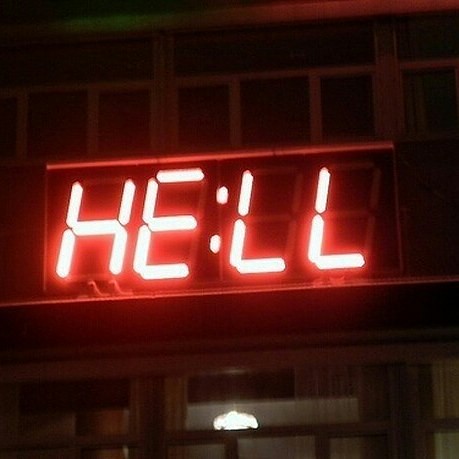This photograph captures a night-time scene outside a building, characterized by low ambient light. Central to the image is a digital sign resembling a clock or timer, prominently displaying the red neon numbers "7734." When viewed upside down, these numbers spell out the word "HELL." The sign, which is perched on a dark shelf-like structure, could easily be mistaken for a timer or an alarm clock. Above this sign are several windows, suggesting it's attached to the side of a building. Below, through a window, an illuminated ceiling light fixture is visible, enhancing the eerie ambiance of the scene. The overall mood is dark and somewhat mysterious, emphasized by the sign's provocative message and the surrounding dim lighting.